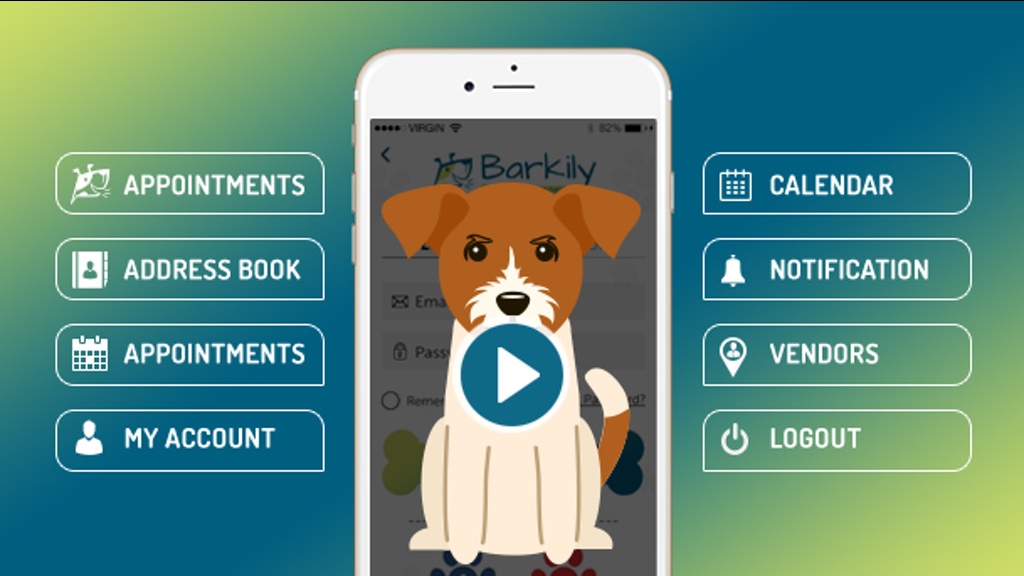This screenshot captures a vibrant web page featuring a prominent central photograph of a cartoon dog with a brown head, white body, and a white-tipped brown tail. A play button is positioned over the dog, indicating a video feature. The photo of the dog is displayed on a phone screen, with a darkened background that includes the word "Barkley." Surrounding the phone image are eight interactive boxes aligned vertically, four on each side. On the left, the options are labeled as Appointments, Address Book, Appointments (again), and My Calendar. On the right, the options include Calendar, Notification, Vendors, and Logout. The background of the webpage transitions through a gradient of yellow to green, then blue, green again, and back to yellow, adding a dynamic and colorful aesthetic to the interface.